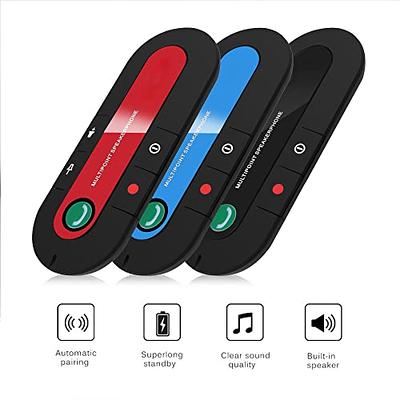A vertical rectangular image with a faint outside border features three black electronic devices with oval shapes, each having differently colored faces: one is red-based, the middle one is blue, and the last one is black. Each device has a distinct green button featuring a half-circle design at the bottom. The devices are likely audio-related and might have additional communication capabilities. Along the bottom of the image, there are four black squares with white interiors, each displaying a unique symbol and a label below, although the text is mostly unreadable. The recognizable icons indicate functionalities such as automatic pairing, volume control, battery charging (labeled "superior on standby"), and clear sound quality, hinting at features like built-in speakers and possibly more. The image is set against a white background.